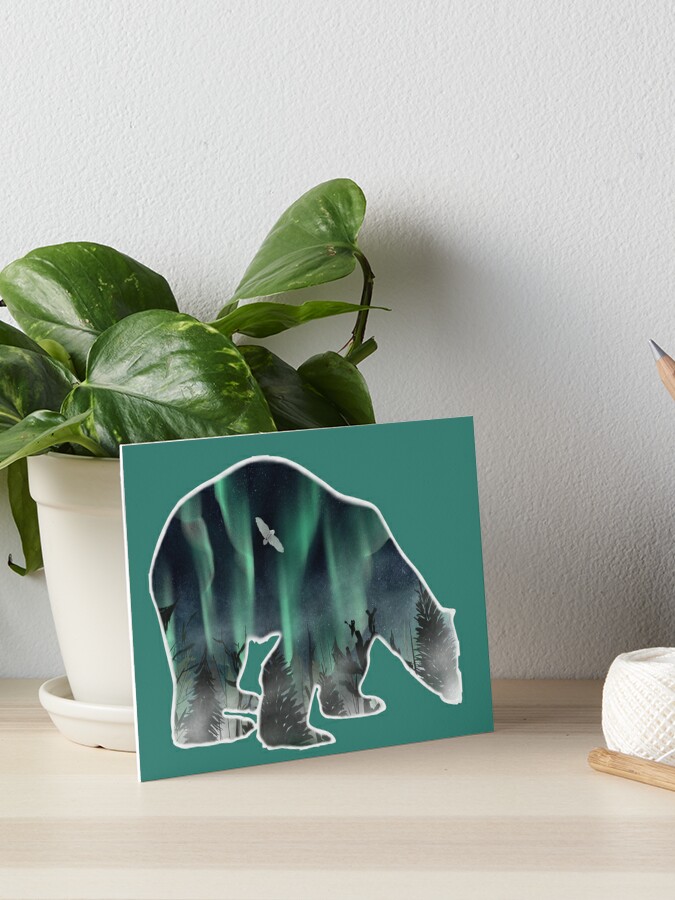The image features a bright, sunlit scene showcasing the top of a light beige wooden dresser against a white wall. Centered on the dresser is a small, vibrant green plant with glossy leaves, housed in a sleek white ceramic planter. Leaning against the planter is a square green card with a white outline of a polar bear. The bear's outline contains a vivid depiction of the aurora borealis, with pine trees visible near the feet and head, and streaks of green light cutting through a dark blue night sky. A white bird, possibly an owl, is also seen flying within the bear’s outline. On the right edge of the dresser, partially visible, is the corner of a candle, adding a touch of warmth to the scene. The overall setting is bathed in natural light, enhancing the clarity and vibrancy of the elements.